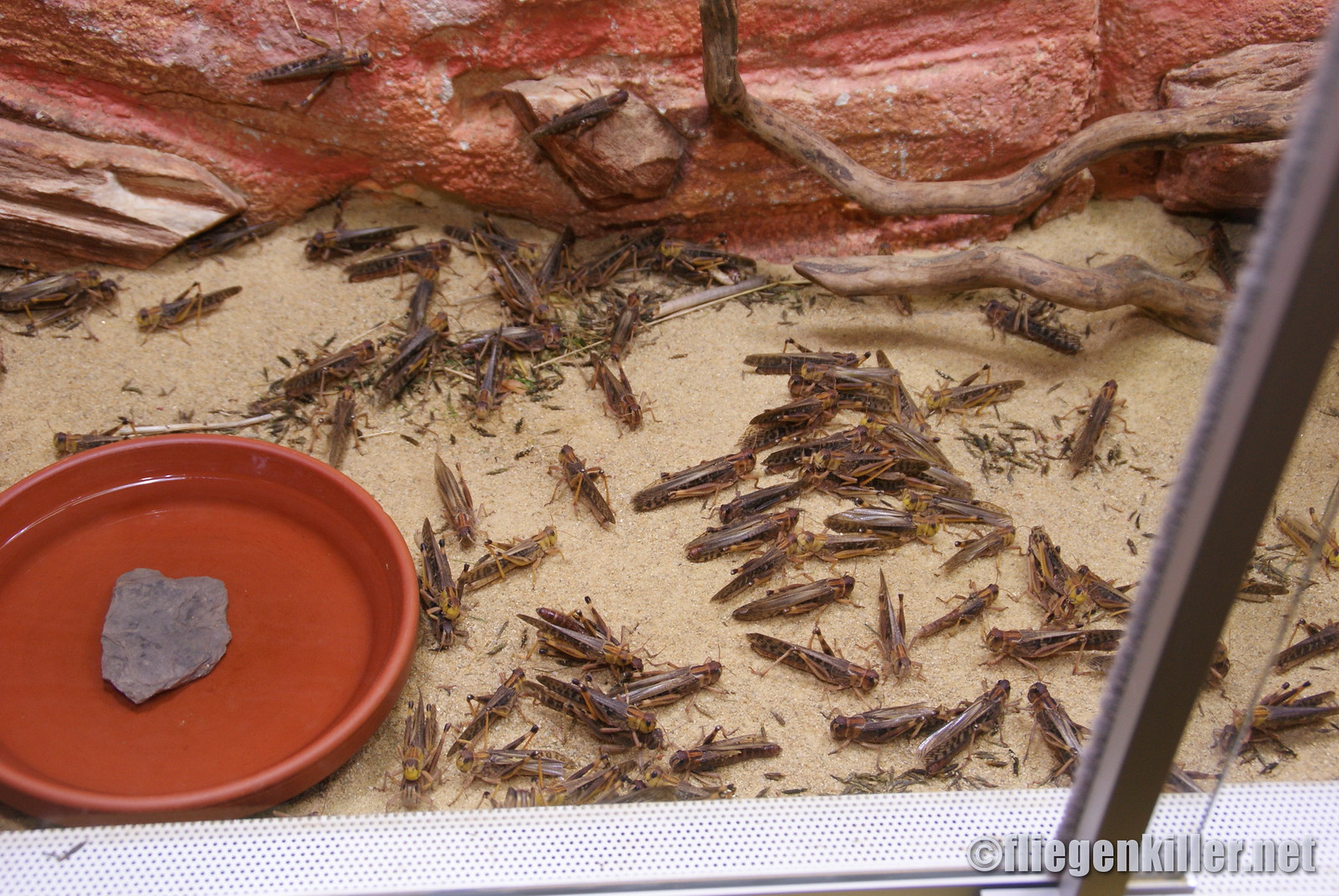The image depicts a bunch of brown roaches, both dead and alive, situated within a red enclosure that appears quite filthy and revolting. The enclosure includes a red bowl with a rock in the center surrounded by a red stone wall, a window providing a view inside, and a grate below. The scene is captured in an unsettling and disgusting perspective, accentuated by the unpleasant presence of these large roaches. The background also displays the text "filegenkiller.net."